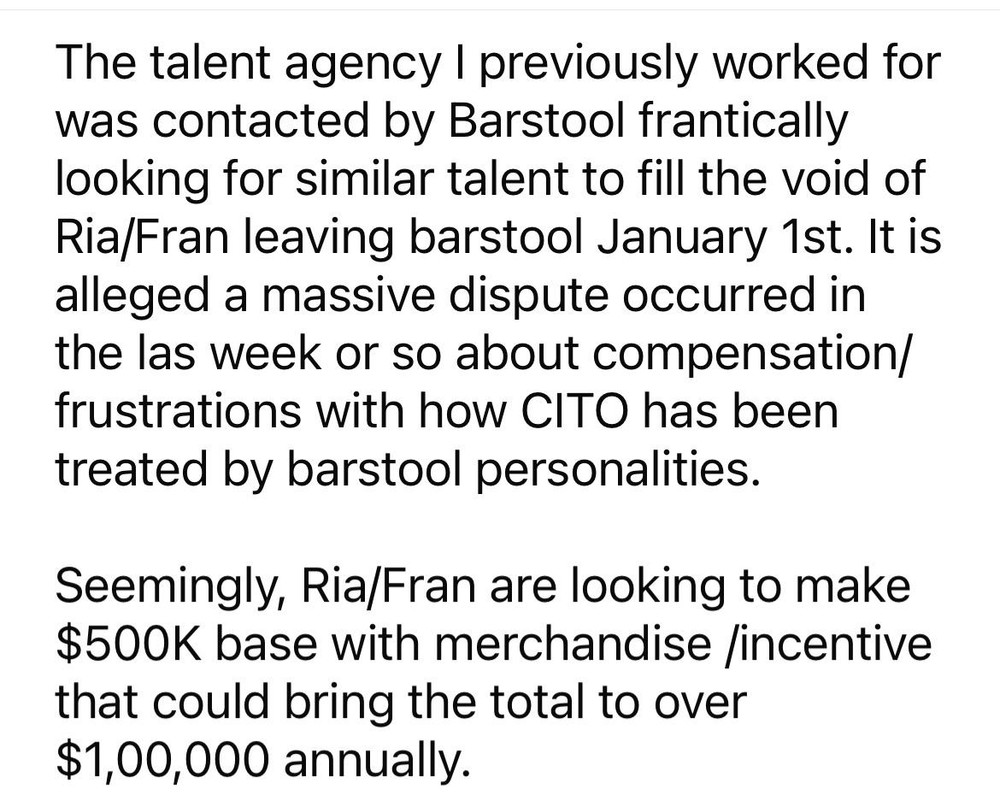The image features a block of black text on a plain white background, resembling content that one might type in a word processing document. The text discusses a situation involving Barstool Sports and a talent agency. According to the message, Barstool Sports urgently contacted the talent agency the person had previously worked for, seeking talent to replace individuals named Rhea and Fran, who are set to leave Barstool on January 1st. The message alleges that a severe dispute arose recently regarding compensation and ongoing frustrations related to how Barstool personalities have treated the "CITO" (Chicks in the Office) show. It is suggested that Rhea and Fran are negotiating for a base salary of $500,000, with additional earnings from merchandise and incentives potentially increasing their total annual compensation to over $1 million. The text appears to contain a numerical typo, as the figure mentioned includes five zeros, while seven zeros seem to be the accurate representation of the intended amount. This statement likely originated from social media, given its speculative nature and style.